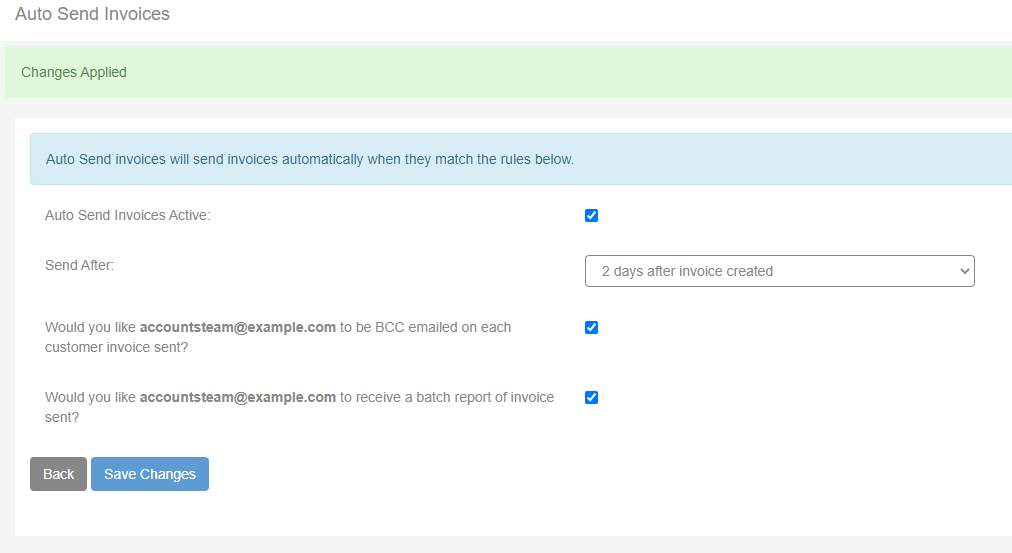The image features a user interface screen for an invoicing application with a primarily white background, containing various labeled sections and action buttons. 

At the top-left corner of the screen, a light green box with green text displays the message "Changes Applied." Directly below, a blue box with white text explains the feature "Auto Send Invoices" with the description: "Auto send invoices will send invoices automatically when they match the rules below."

The rules listed are as follows:
1. "Auto Send Invoice Active" which is marked with a blue check sign indicating it is enabled.
2. "Send After" featuring a dropdown menu on the right that specifies "2 days after invoice created."

Further options include:
- "Would you like accounts.team@example.com to BCC email on each customer invoice sent?" which is also marked with a blue check sign, confirming it is enabled.
- "Would you like accounts.team@example.com to receive a batch report of invoices sent?" similarly indicated with a blue check sign, confirming it is enabled.

At the bottom-left of the image, there are two action buttons. The first button labeled "Back" is gray with white text. To its right, the "Save Changes" button is blue, also featuring white text.